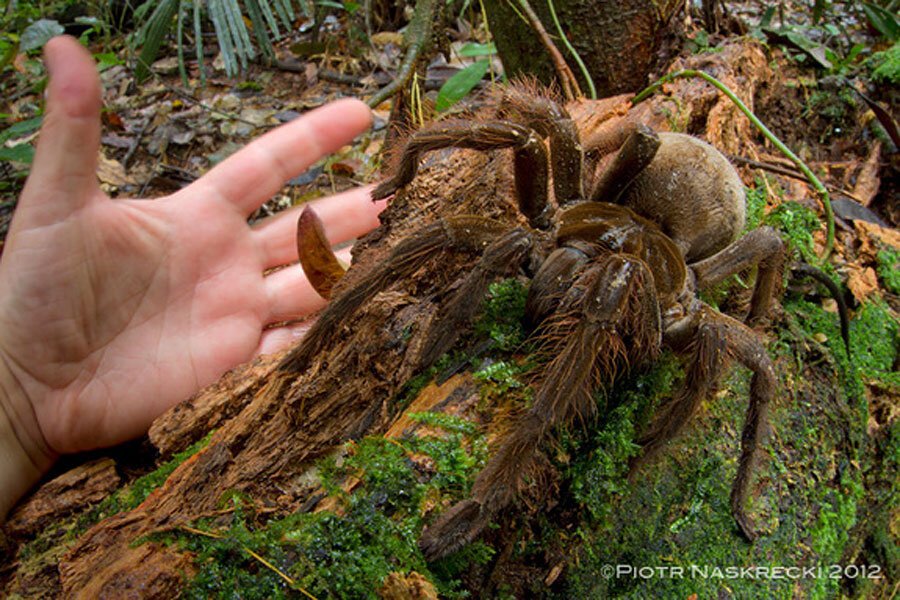This outdoor daytime photograph captures an enormous, brown and furry tarantula, likely a Goliath bird eater, perched on a decaying, moss-covered log that begins at the lower left and right corners and extends toward the upper right. The log, festooned with vibrant green moss, contrasts with various leaves, sticks, and flora typical of a rainforest setting. To the left of the tarantula and log, a Caucasian man's left hand, palm up and fingers spread, highlights the spider's immense size, which appears even larger than the hand itself. The photograph, which seems to be taken in a moist environment, includes a copyright mark in the lower right corner with the text: © Piotr Naskrecki 2012.